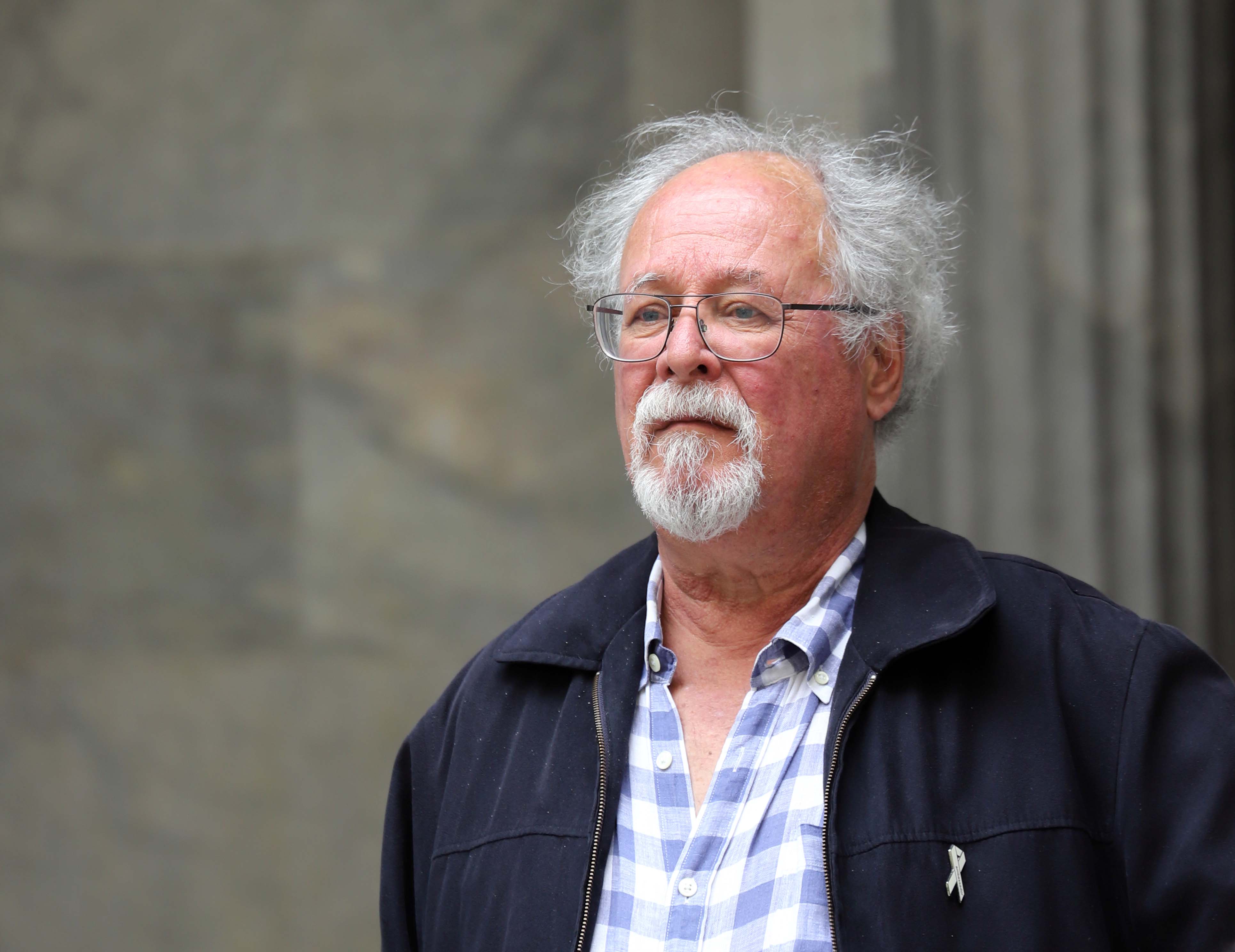This is an indoor photographic image of an older Caucasian man, seemingly in his 60s, with a weathered, contemplative expression. He is balding, with a fringe of uncombed, wispy gray and white hair around the sides and back of his head. His facial hair includes a gray and white mustache and goatee, which is more neatly trimmed. He wears square wireframe glasses reminiscent of the 70s or 80s, which frame his blue eyes. His skin appears slightly reddish, possibly windburned.

The man is dressed in a dark navy zip-up jacket with a collar, adorned with a small white ribbon on the left side, and a blue and white plaid button-up shirt, unbuttoned at the top to reveal bare skin underneath. He is looking slightly to the lower left, away from the camera, adding to his reflective demeanor.

In the background, there is a gray marble or stone wall and a pillar, suggesting he might be near a monument or a significant structure. The overall scene evokes a sense of solemnity and introspection. The image is devoid of any text.